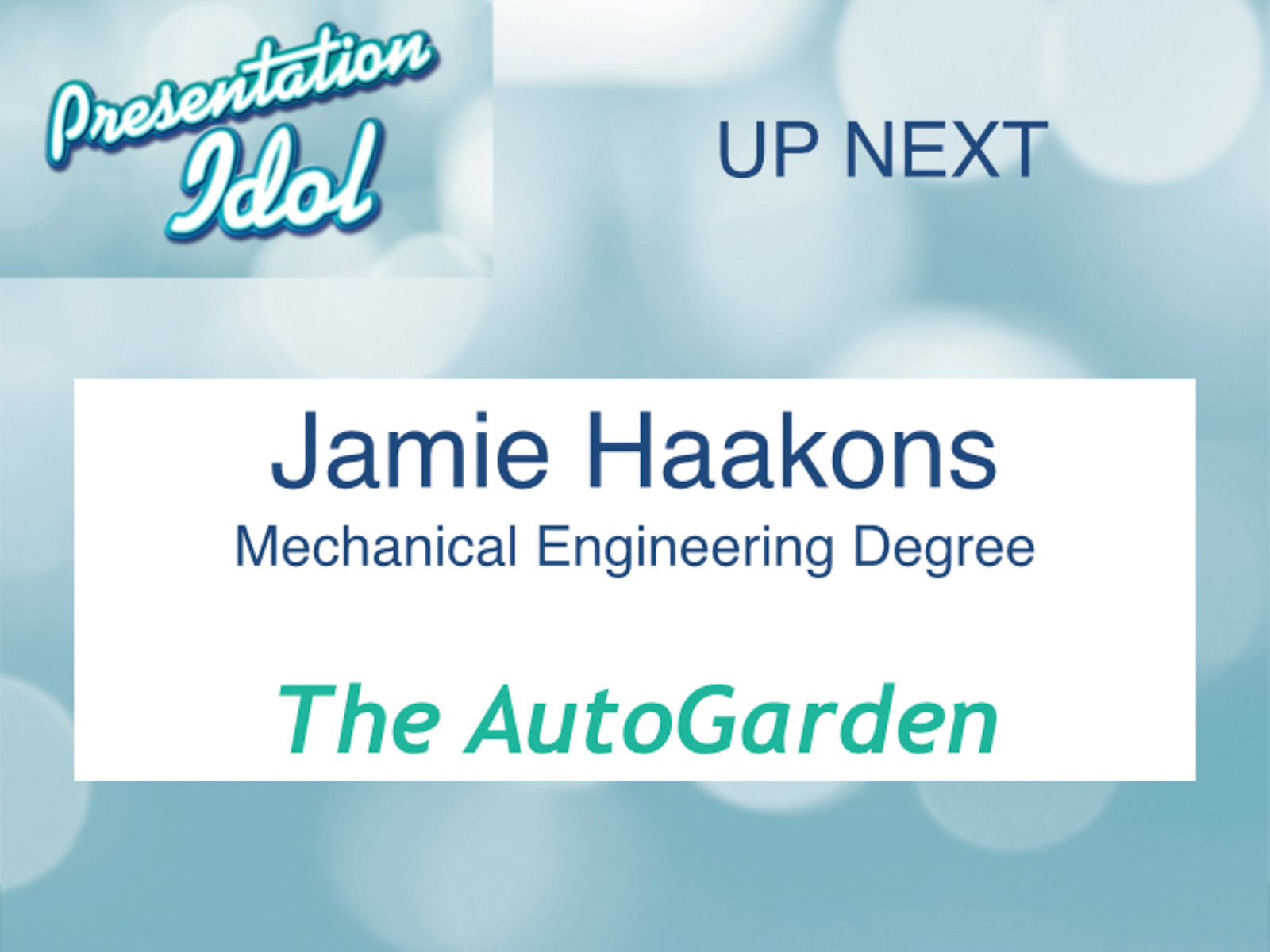The image is a landscape-oriented slide with an abstract aqua blue background and out-of-focus white circles, giving it a glossy, shiny appearance. In the upper left corner, there is a logo similar in style to the American Idol logo, reading "Presentation Idol" in white script with a navy drop shadow. Adjacent to it on the right, in dark blue text, it says "Up Next." Dominating the center of the slide is a large white rectangular text box. At the top of this text box, in dark blue font, it reads "Jamie Haakons' Mechanical Engineering Degree." Below that, in italicized teal lettering, it says "The Auto Garden." The slide appears to be part of a presentation, perhaps an introductory or transitional one announcing the next speaker and the topic of their presentation.